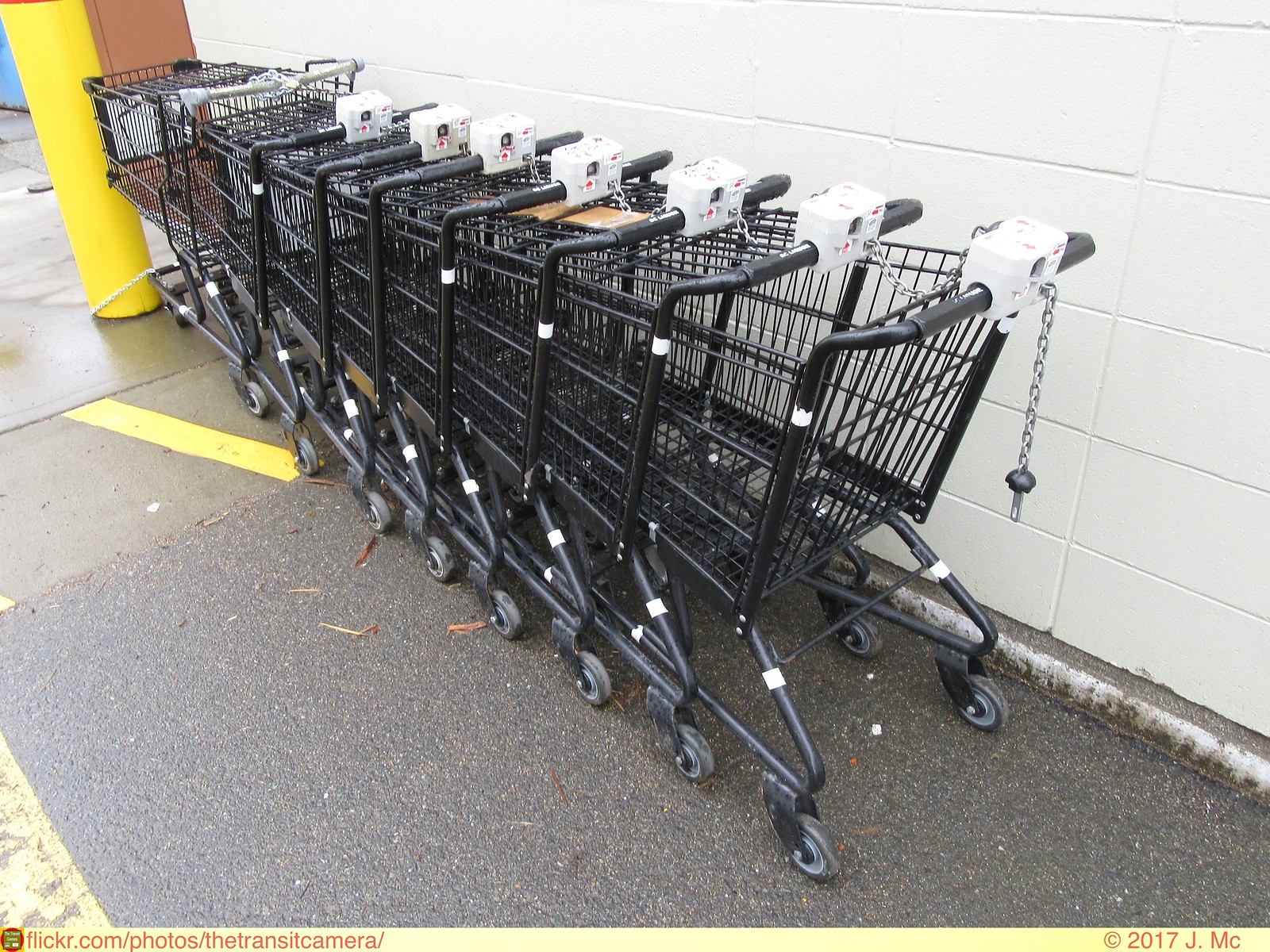This outdoor photograph captures a row of 8 to 9 black shopping carts neatly stacked together against a large, partially visible white brick wall, presumably outside an Aldi supermarket. The shopping carts are secured with a theft deterrent system, requiring a quarter to release each cart, identifiable by the chain mechanisms on their handles. At the front of the row, in the top left corner of the image, stands a prominent yellow pole, which also has a rope tied around it. The pavement transitions from yellow-lined concrete to plain asphalt, suggesting a walkway leading into the store. The ground appears wet, hinting at recent rain. At the bottom right of the photo, a web address reads "flickr.com/photos/thetransitcamera," followed by a "© 2017 J.MC" watermark.